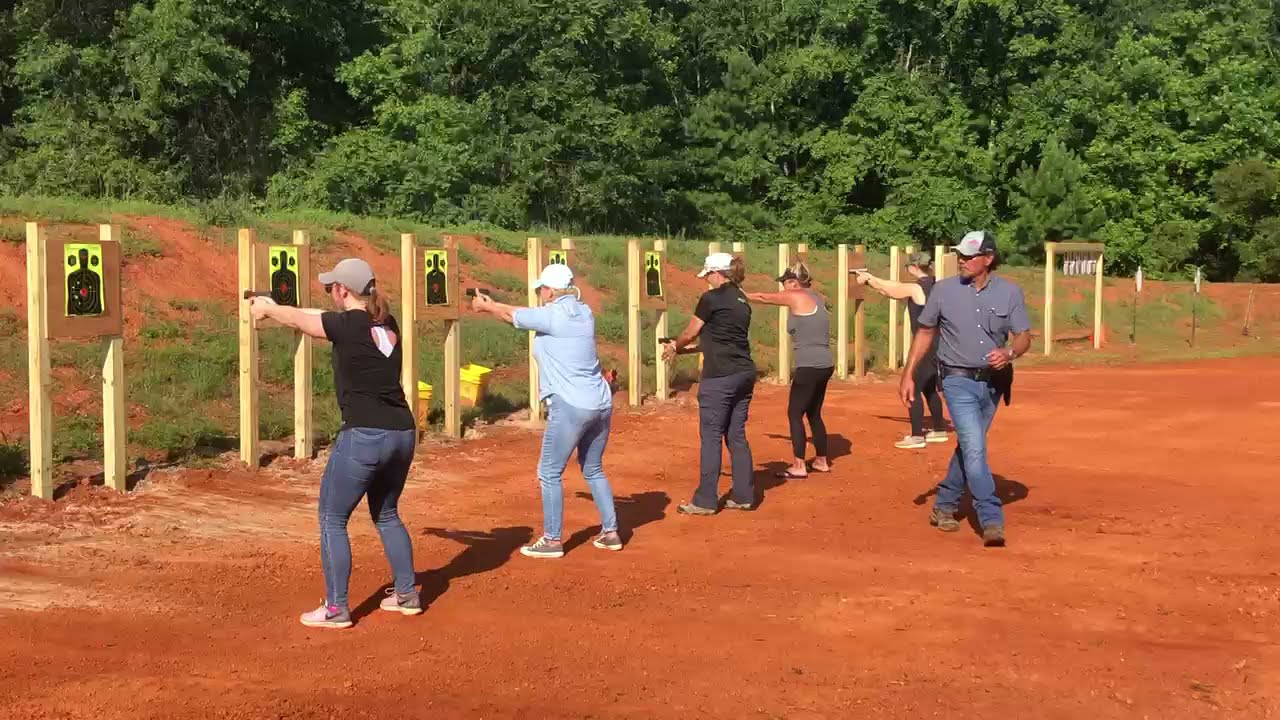At an outdoor shooting range, five women, all wearing hats, stand on reddish-orange dirt and aim their guns at yellow shooting targets. These targets depict black human silhouettes with red bullseyes at the chest and are mounted on plywood boards held up by wooden poles. The range is bordered by a slope covered with patches of grass and more of the orange-brown dirt, leading up to a dense backdrop of dark green trees. On the right side of the image, a male shooting instructor, distinguishable by his white and black baseball cap, gray collared shirt, blue jeans, and brown boots, walks towards the women, attentively observing and offering guidance. The woman in the middle of the group has her gun lowered, while the others maintain their aim.